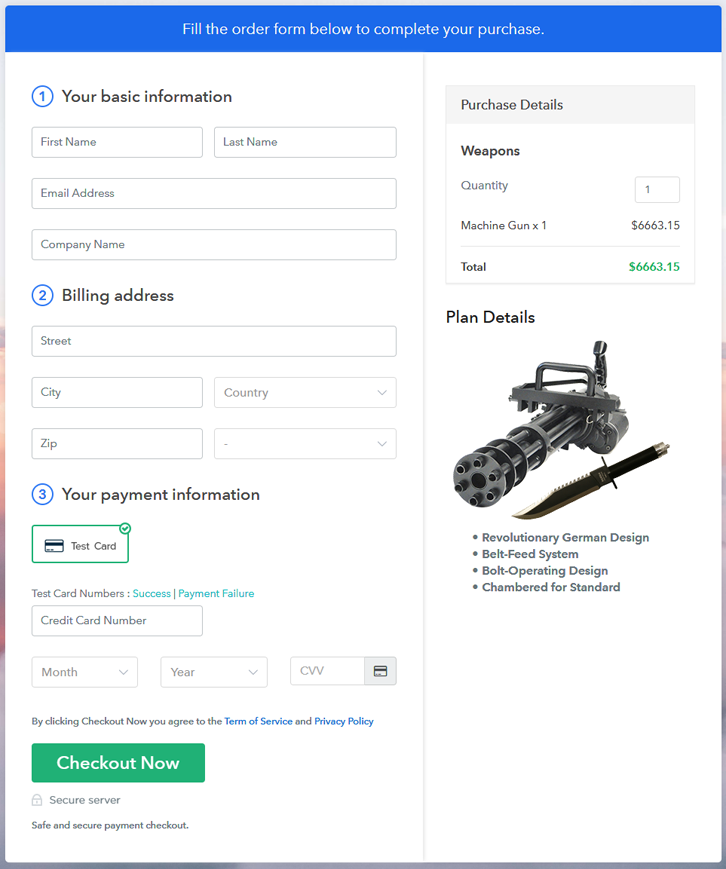The image displays a purchase completion form on a retail website, structured with a prominent blue header at the top that reads, "Fill the order form below to complete your purchase." The form itself is divided into several sections for user information input.

1. **Your Basic Information:**
   - Boxes are provided for Full Name, Last Name, Email Address, and Company Name.

2. **Billing Address:**
   - Fields include Street, City, Country (with a dropdown selection), Zip, and another unspecified dropdown box.

3. **Your Payment Information:**
   - There are fields for Test Card, Test Card Numbers, and dropdown menus for Month, Year, and CVV.

Beneath these sections, a prominent green button labeled "Check Out Now" is visible.

On the right side of the form, under the heading "Purchase Details," the summary includes:
- **Item:** Machine Gun
- **Quantity:** 1
- **Price:** $6,663.15 each
- **Total:** $6,663.15

Below this, under "Plan Details," there is an image of the machine gun referenced in the purchase summary.